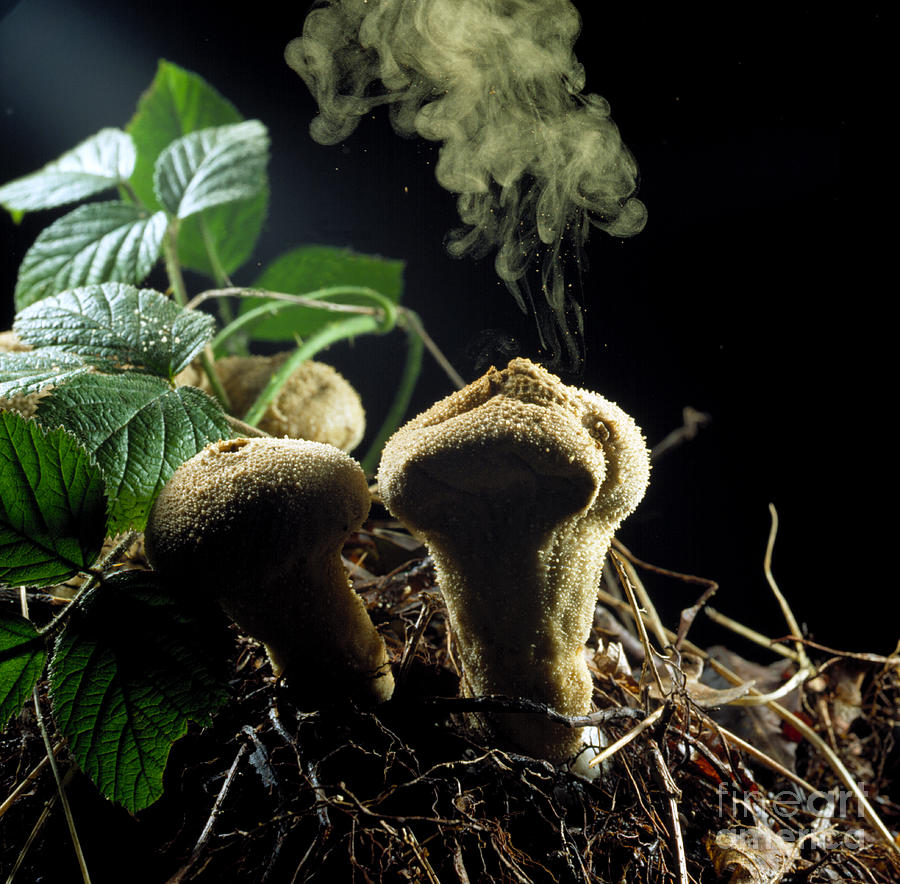In this captivating real-life photograph, the central focus is on a peculiar botanical specimen that resembles a mushroom but exudes an almost creature-like presence. The organism, with its distinctive mushroom shape, features a leathery surface that appears to have tiny, fur-like textures. The image captures two such entities emerging from a substrate littered with twigs, dead grass, and leaves, reminiscent of a compost pile.

The organism on the right is particularly intriguing, as a plume of smoke billows from a small opening at its top, giving the impression that something has just been expelled. In contrast, the organism on the left retains a more traditional mushroom-like form with a plain, undisturbed hole at its apex. The one on the right, however, shows signs of breaking apart at the top.

Surrounding the mushroom-like structures are green leaves that closely resemble mint leaves, characterized by their leathery texture. Behind these leaves, spiky vines intertwine with dead vines, adding to the complex layering of the scene. The backdrop is a deep black, with beams of light slicing through and illuminating the tops of the mysterious organisms. This interplay of light and shadow creates a stark contrast, accentuating the beige, khaki-colored tones of these enigmatic, mushroom-like formations.